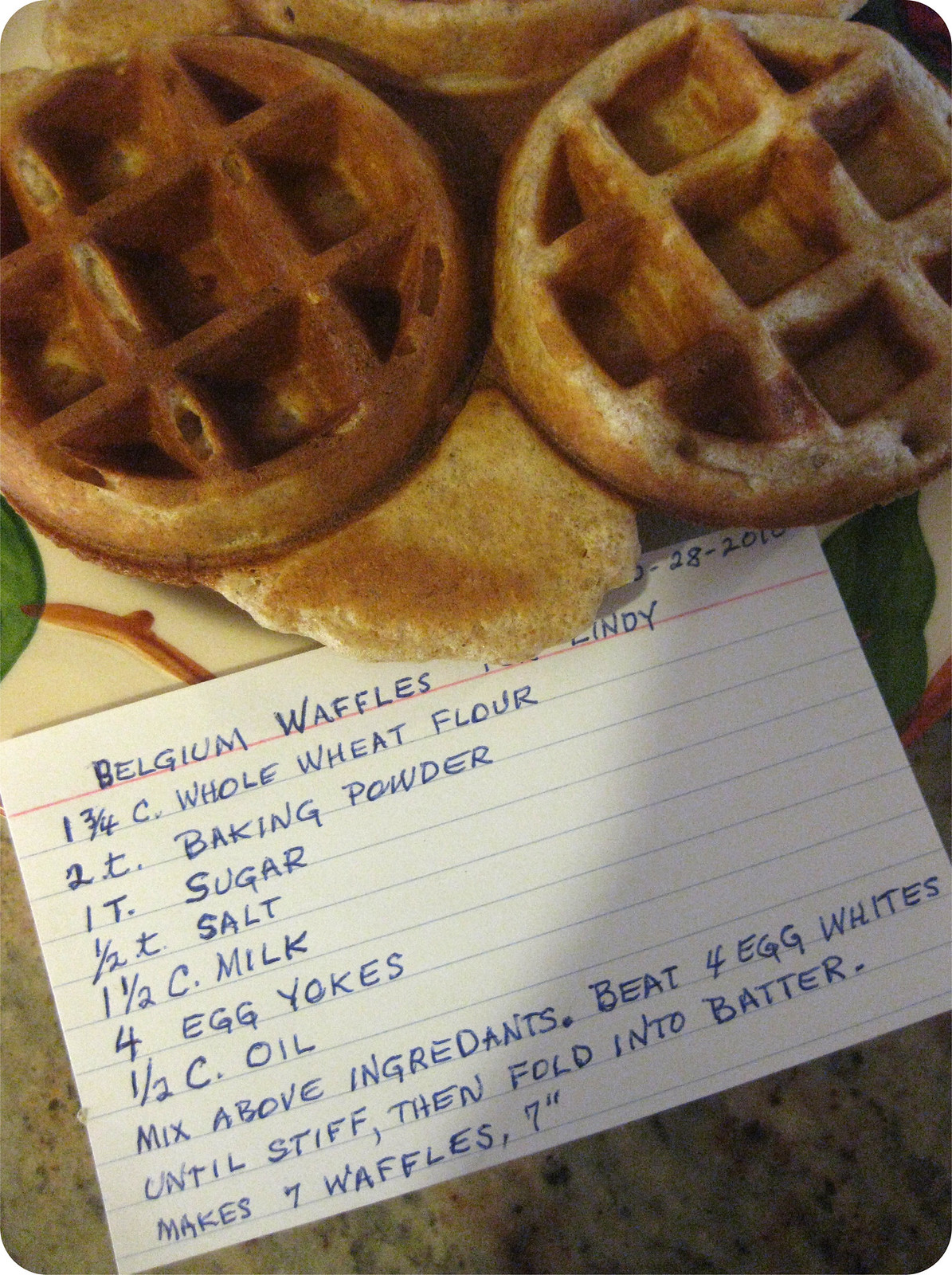The image shows a handwritten recipe on an ordinary white index card with blue lines and blue handwriting, partially covered by two Belgian waffles drizzled with syrup, likely maple syrup. The recipe beneath the waffles lists the ingredients and instructions for making Belgian waffles. Specifically, it calls for one and three-quarters cups of whole wheat flour, two teaspoons of baking powder, one tablespoon of sugar, half a teaspoon of salt, one and a half cups of milk, four egg yolks, and half a cup of oil. The instructions instruct to mix these ingredients, then beat four egg whites until stiff and fold them into the batter, yielding seven seven-inch waffles. The waffles sit atop a plate on a dark surface, adding to an overall feeling of a cozy breakfast setup.